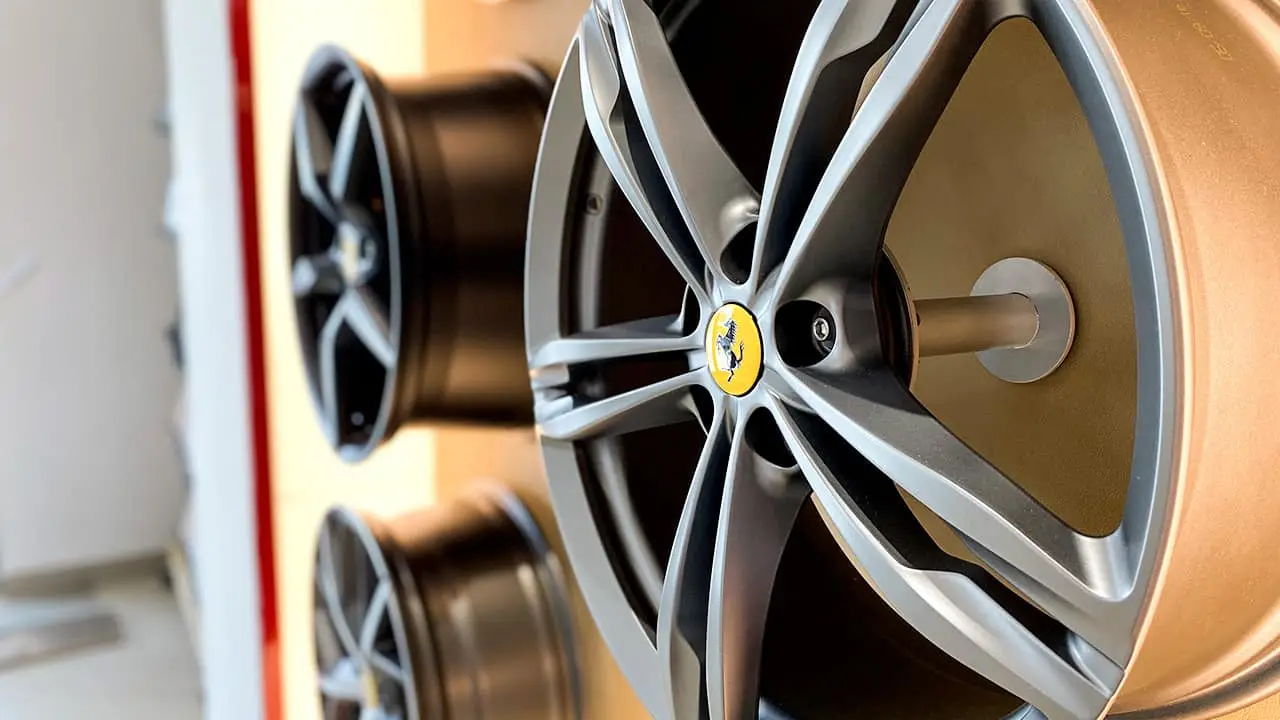The image depicts three automobile rims suspended on a wall. The rims are primarily metallic, with the most prominent one in the foreground exhibiting an orangey-gold hue with silver spokes and a distinctive yellow centerpiece that features an emblem resembling a rearing horse, reminiscent of a Ferrari logo. The other two rims, positioned further back and slightly blurred, appear to have a coppery color with similar silver spokes and yellow centerpieces. The wall behind the rims is a gradient of orange to yellow, with a thick, uneven white squiggly line on the left side and a red stripe extending vertically. The lower left portion of the background transitions to a blue-gray color with gray splotches. The room where the rims are displayed is well-lit, but otherwise nondescript.